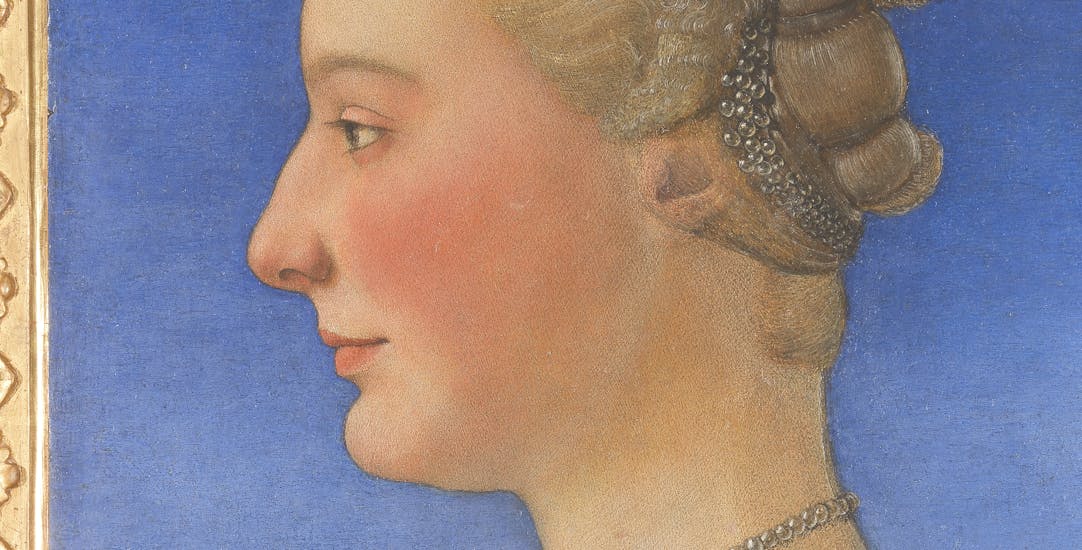This detailed medieval-style portrait depicts a woman’s side profile against a bright sky blue background. Her fair skin contrasts with her large nose, pronounced chin, flushed cheeks, and striking blue or golden-brown eyes. Her pink lips are slightly smiling as she gazes off into the distance, her face framed by her intricate updo. Her blondish-grayish hair is elaborately styled, sweeping away from her face into a braid or bun adorned with pearls and possibly sparkling silver hair jewelry. She also wears a string of pearls around her neck. The light blue background is bordered on the left by a painted golden frame, adding a touch of regality to the composition.